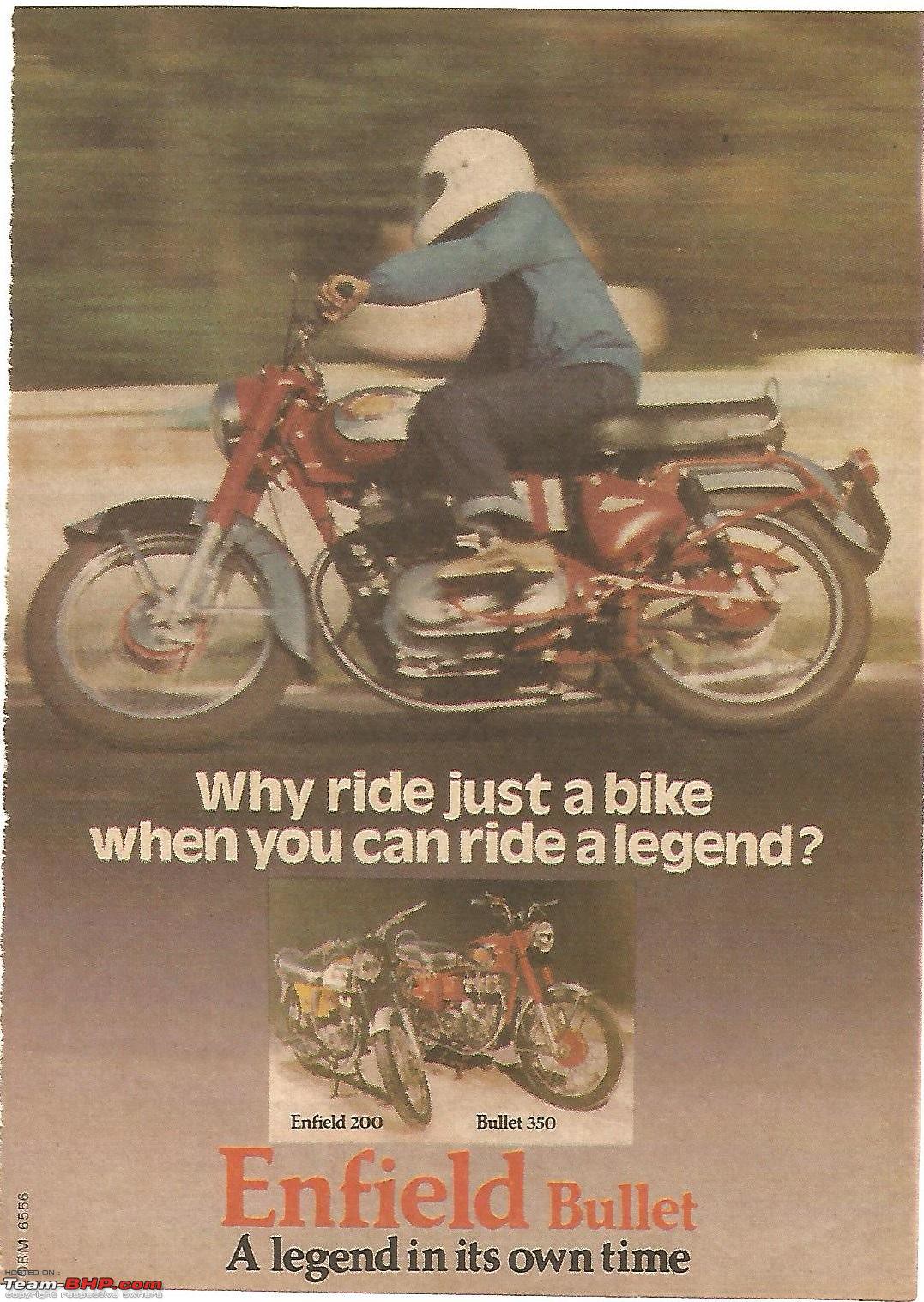The advertisement features a person riding a classic red motorcycle with silver details, captured in a dynamic, fast-moving background. The rider is dressed in a cyan (or light blue) jacket, white helmet, jeans, and yellow shoes, and is turning to their right. The image itself has a grainy, vintage feel. Below the main image, in white text, is the phrase, "Why ride just a bike when you can ride a legend?" Accompanying this message is a photo of two motorcycles: the Enfield 200 on the left and the Bullet 350 on the right, both appearing in what looks like a showroom. Below this photo, the text reads, "Enfield Bullet, a legend in its own time." In the lower right corner, the watermark TeamBHP.com is faintly visible.